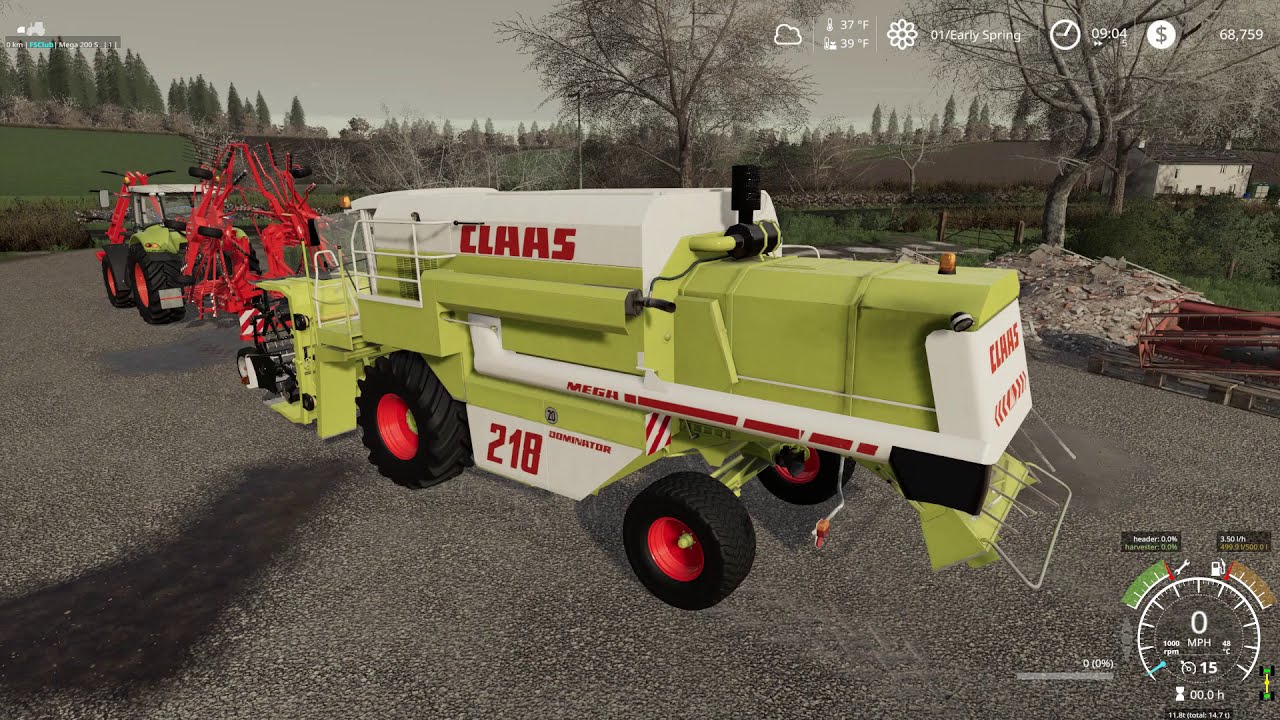The image displays a vividly detailed, video-game screenshot set outdoors on a gravel-textured pavement. Central to the scene are two prominently featured construction utility vehicles. The primary vehicle, positioned centrally, is a pale green and white truck with large tires and red lettering spelling "CLAAS" along with the number "218" near the tires. To its upper left, a red bulldozer-like tractor with equally large tires complements the scene. The setting extends to show several dead trees in the middle and upper right, contrasting with patches of vibrant green grass and healthy-looking trees to the upper left. Above, in a partly cloudy sky, weather indicators and different types of gauges, including a miles-per-hour gauge set to zero, hint at the game's interface. The color palette includes shades of black, gray, green, red, white, and light blue, enriching the scene with diverse but coherent tonal elements.